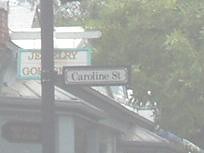A small, blurry image captures a scene with several prominent features. In the background, a dense cluster of green trees can be seen, providing a lush backdrop. A large house, adorned with several white posts along its front, stands prominently in the mid-ground. A tall telephone pole is positioned near the house. Attached to this pole are two signs: the upper one is white with a large black circle and some lettering within it, while the lower sign is white bordered in black with black text. Above the treeline, a sliver of blue sky peeks through, adding a touch of contrast to the verdant surroundings.